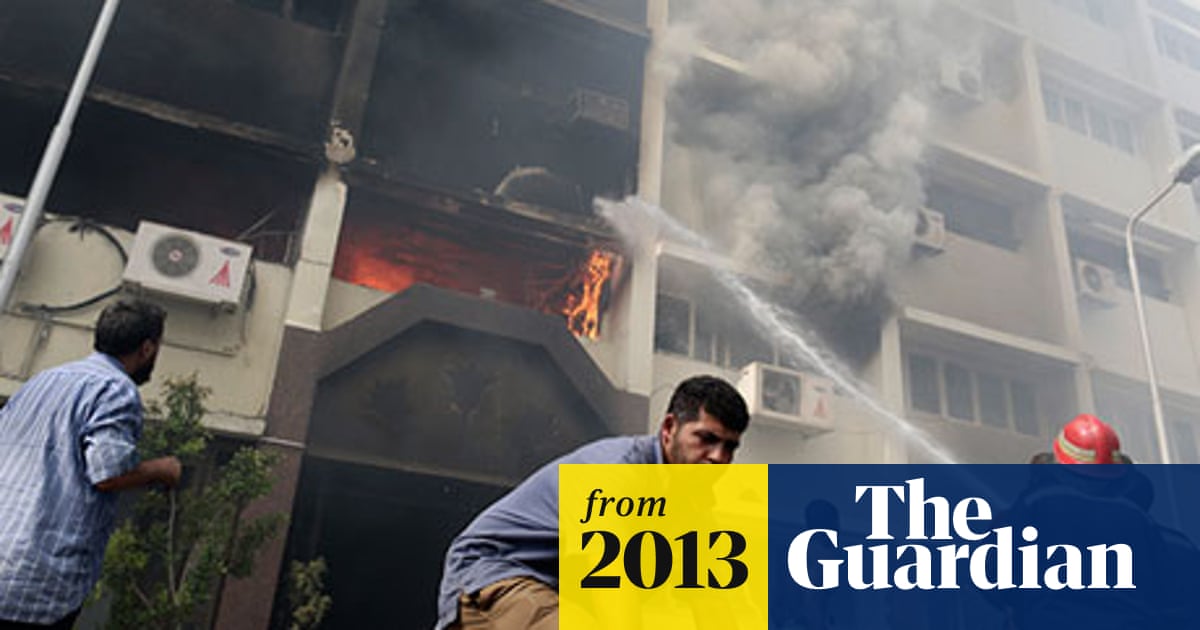The image, appearing to be a header for a 2013 article from The Guardian, captures a dramatic scene of a burning apartment complex, possibly from the 1970s. The fire, raging and intense, has engulfed multiple floors within the same column of the building, leaving the left side blackened with ash and billowing smoke, while parts of the right remain off-white. Flames are visible through several windows. In the foreground, a man in a blue shirt and beige pants, with dark hair and possibly a beard, bends down near a firefighter who is aiming a hose at the fire. Another man in a blue and white striped shirt is seen looking up at the blaze. The Guardian's distinctive yellow, blue, and white banner, located at the bottom right corner of the image, prominently features "From 2013" in black letters on a yellow background, and "The Guardian" in white letters on a blue background. The scene is chaotic, filled with action and urgency as firefighters and onlookers confront the spreading inferno.